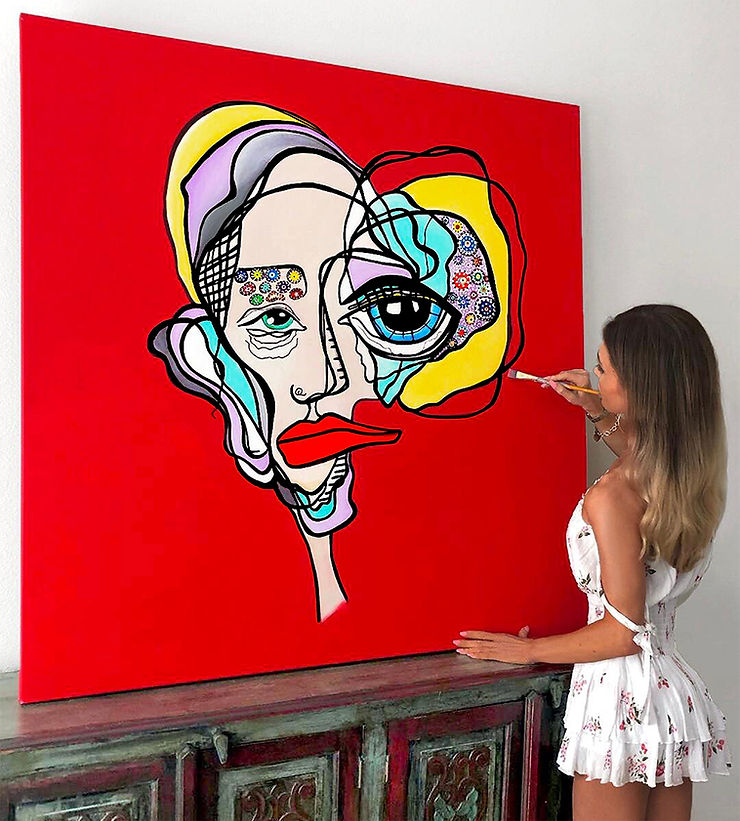In the image, a woman is intensely focused on a large painting with a red background that spans high up the wall. She is wearing a very short white dress adorned with a floral print, and a ribbon or bow is wrapped around her left arm. Her hair cascades down to the middle of her back, dark brown at the top and gradually lightening to a dirty blonde at the tips, suggesting it has been dyed. She is using her left hand to steady herself against a wooden cabinet or shelf, and she holds a paintbrush dipped in red paint in her right hand. The painting she is working on features an abstract face characterized by asymmetrical shapes: large, exaggerated blue eyes, one possibly adorned with small gears or flowers, a crooked nose, a thin neck, and big red lips. The face also features a variety of colorful elements like a head covering in yellow and gray and ear details in blue, white, and gray ovals. Despite her deep engagement with the art, there is a sense of ambiguity as to whether she is actively painting or simply posed to appear so.